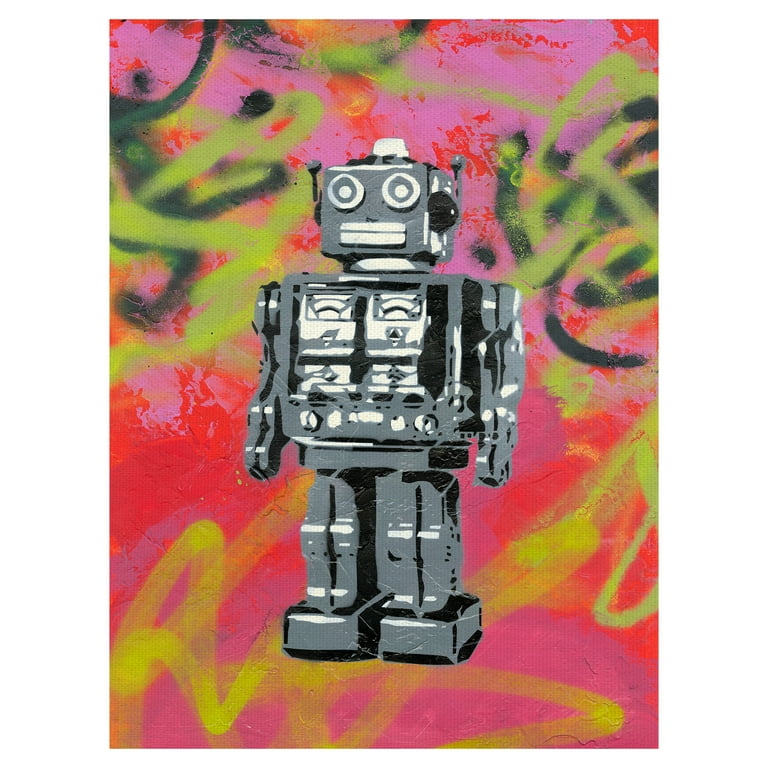The image depicts a tall, narrow painting with a vibrant, graffiti-esque background marked by an abstract layer of red, pink, yellow, and shades of green, blended together through squiggles and spray-painted shapes. Dominating the center of the piece is a retro-styled robot, rendered in shades of gray, black, and white with noticeable stenciling. The robot features distinct, large round eyes with white rims and gray circles inside, each accented by a white dot, giving it a mechanical, yet expressive, visage. It has a square head capped with a white piece and flanked on either side by handle-like structures reminiscent of slot machine levers that may represent antennas. The robot's wide metallic mouth and rigid steel arms, marked by white sections at the shoulders, elbows, and wrists, convey a classic, almost antiquated robotic aesthetic. Its chest displays a series of white and gray elements resembling tape decks or wheels, and its legs terminate in square, metallic shoes. With its blocky stance slightly angled to the left, the robot adds a pronounced contrast to the chaotic and richly hued backdrop.